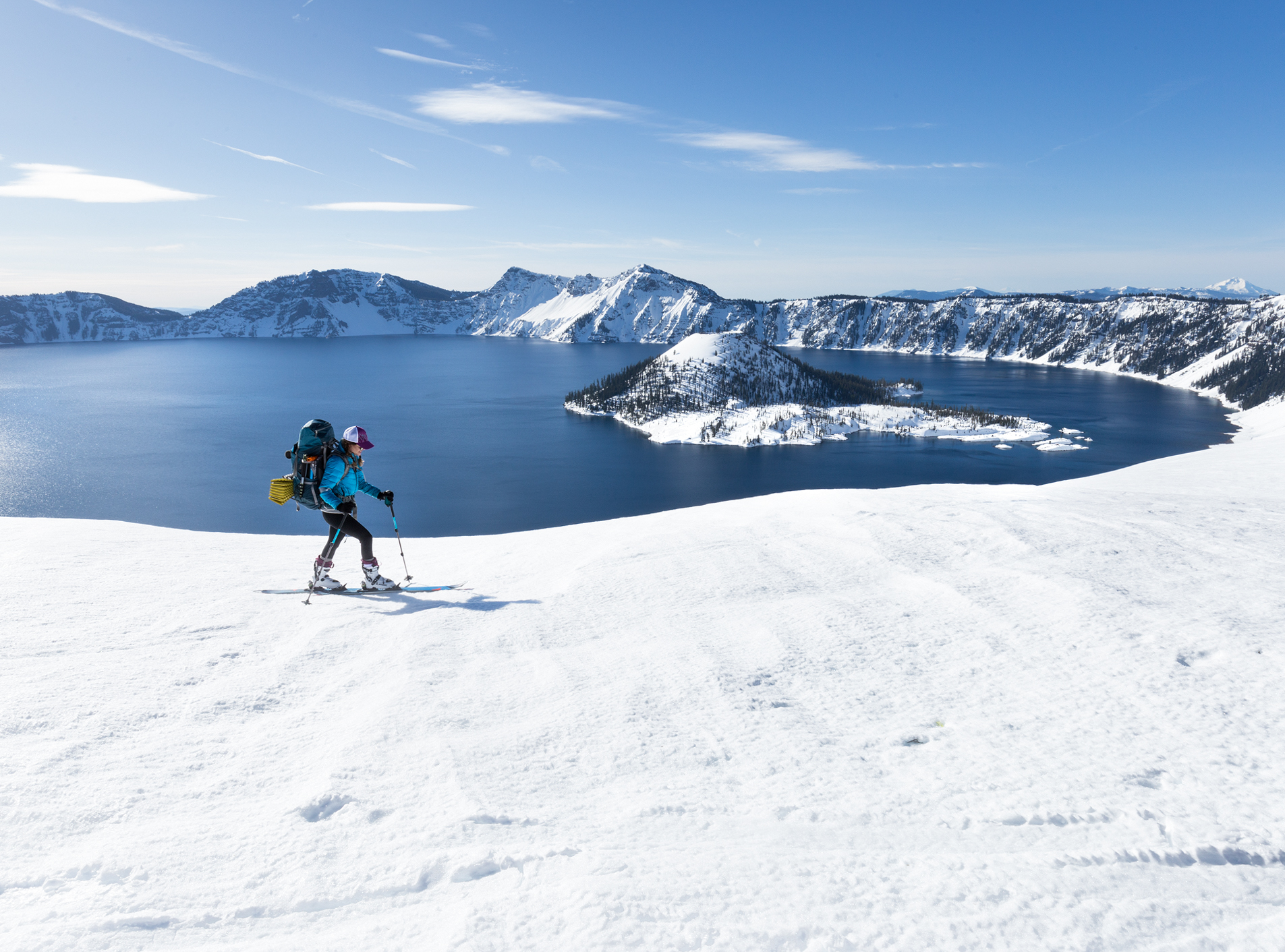A panoramic, wide-angled photograph captures a breathtaking winter adventure. Centered in the image is a woman traversing a snow-covered landscape on skis. She is dressed in a distinctive ensemble featuring a cyan blue heavy jacket, dark blue pants, black gloves, and a gray undershirt. A purple-front and white-back baseball cap sits atop her head, while her feet are secured in white, thick ski boots with a purple lining. She carries a large, stuffed blue backpack with black compartments, and a yellow canister stands tall on her back. She uses two poles for balance.

Her shadow falls to the right side on the pristine white snow that winds around the terrain. To her left, a vast, unfrozen lake is nestled among a majestic, snow-capped mountain range. Evergreen trees line parts of the lake, creating a picturesque contrast against the snow. Overhead, the sky is a vibrant blue, adorned with scattered clouds, setting the scene under clear daylight. This photograph eloquently captures the essence of a serene and adventurous day in a stunning mountainous winter landscape.